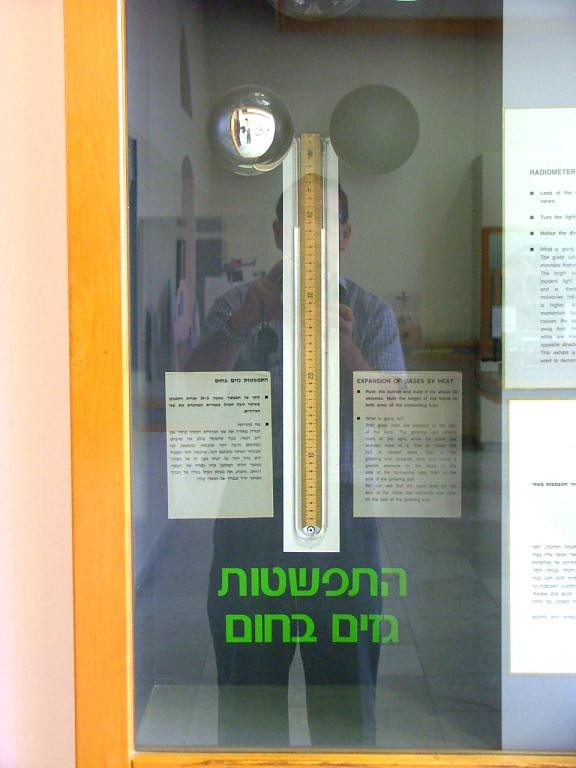The image depicts a glass display showcasing two sheets of paper with handwritten notes, positioned side by side. At the top of the display, there are two spherical objects — one silver and one gray. Between these spheres lies a long, brown ruler, with green writing at the bottom. The glass reflects a person in a blue shirt, seemingly capturing a photo of this arrangement. 

Surrounding the display is an orange trim, complemented by a light pink border. Both the left and right sides of the display feature additional sheets of white paper with black handwritten text. Notably, one of the sheets on the right side prominently displays the word "radiometer" among other inked annotations.